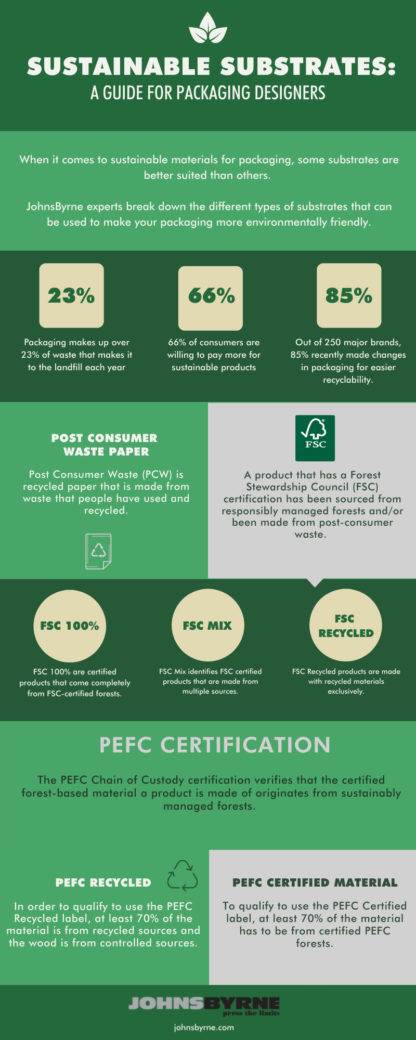This tall infographic, titled "Sustainable Substrates: A Guide for Packaging Designers" by Johns Burn, is designed to educate packaging designers on environmentally friendly materials. The background is divided into sections with varying shades of green and beige, along with smatterings of light grey, and uses white text for clarity. 

The top section reads, "When it comes to sustainable materials for packaging, some substrates are better suited than others." It introduces the theme, emphasizing that the choice of substrate can significantly impact sustainability.

The next section presents key statistics: 23% of all waste in landfills comes from packaging, 66% of consumers are willing to pay more for sustainable products, and 85% of 250 surveyed major brands have recently changed their packaging to enhance recyclability.

Following this, the infographic details various certifications and types of sustainable substrates. One segment explains post-consumer waste paper (PCW) as recycled paper derived from previously used and recycled materials. Another emphasizes the Forest Stewardship Council (FSC) certifications: FSC 100% ensures products come entirely from FSC-certified forests, FSC Mix indicates a combination of sources, and FSC Recycled denotes exclusive use of recycled materials.

Further down, the PEFC certifications are addressed. The PEFC Chain of Custody Certification guarantees that forest-based material comes from sustainably managed forests. The section is split to describe PEFC Recycled, which requires at least 70% of the material to originate from recycled sources, and PEFC Certified, which also mandates that at least 70% of the material be certified by PEFC.

The infographic is visually structured to guide viewers from top to bottom, with each section carefully explaining the importance and criteria of sustainable packaging materials.